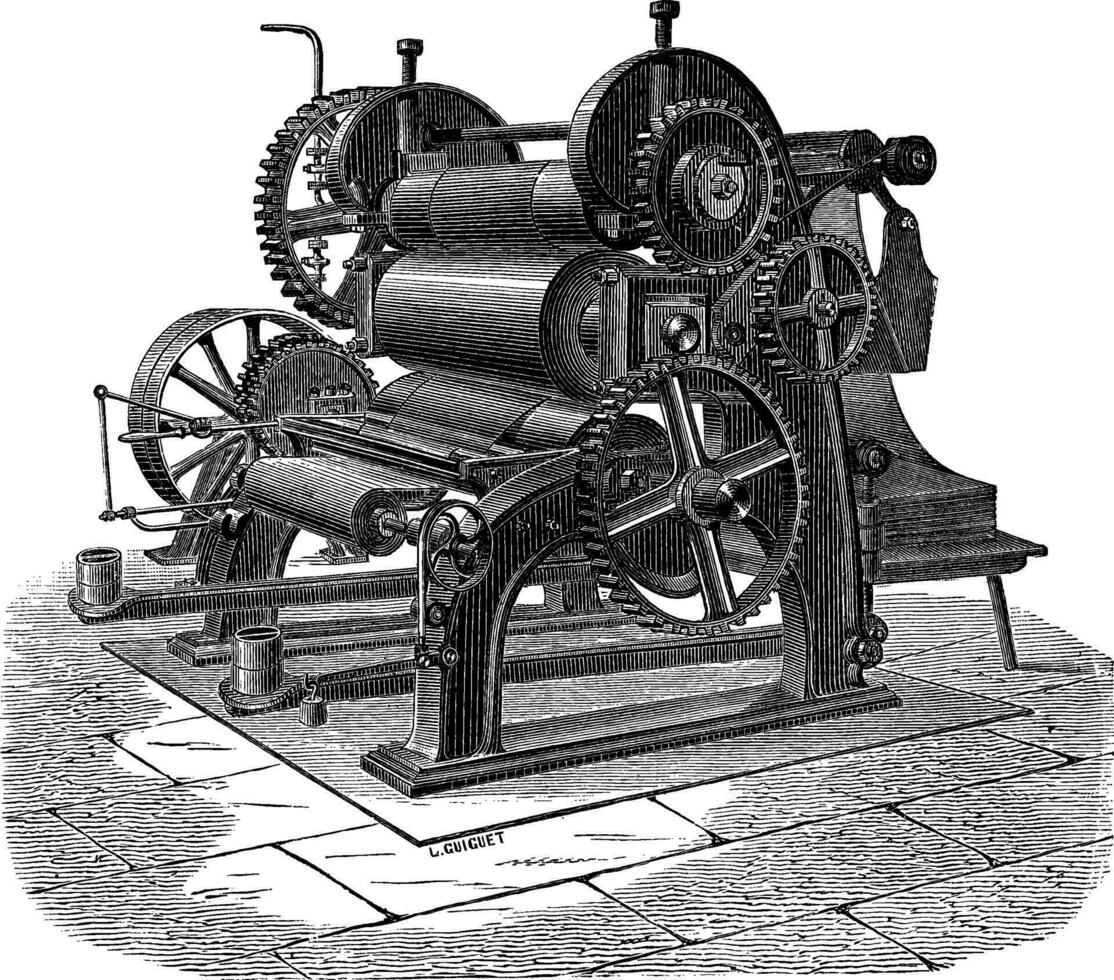This is a black-and-white sketch illustration of an old-fashioned mechanical press, possibly from over 100 years ago, signed by the artist LGK, or Ku Nguit, as faintly indicated on the stone floor below it. The detailed drawing, filled with intricate hash marks, showcases a machine composed primarily of metal, featuring numerous gears, pulleys, and rollers. These elements suggest it might be an automatic loom, sheet metal press, or roller press. The large gears prominently displayed in the foreground interconnect to drive the rollers, while smaller protruding objects that resemble dials might be for adjusting the speed or thickness of materials processed through the press. The press sits on a tiled cement-like floor, with no people present, making the machine the sole focus of this almost square-shaped antique rendering.